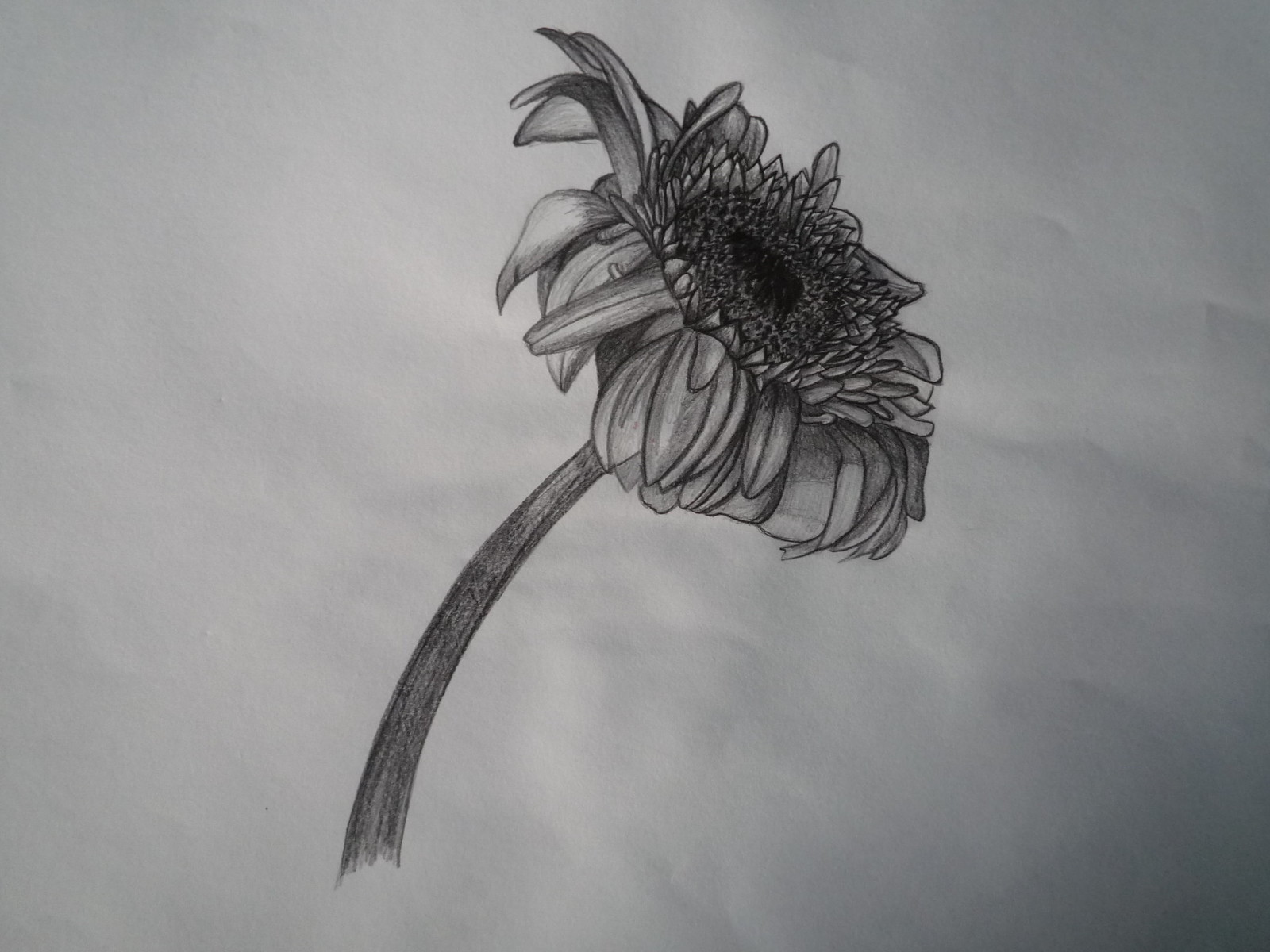This detailed charcoal drawing captures the elegant form of a sunflower, rendered on a slightly wrinkled white or gray drawing pad. The shadow in the lower right-hand corner adds depth to the composition. Starting from the left-hand side, the sunflower's sturdy stem rises toward the center of the artwork, leading up to the full bloom. The sunflower's face is oriented towards the upper right corner, with its leaves elegantly curled downward. The petals of the sunflower display a naturalistic curl, with some gracefully turning down at the edges. The dark black center of the sunflower is surrounded by a lighter halo, providing a striking contrast. Petals radiate from the center, some pointing straight up while others cascade downward, enhanced by delicately drawn shadows that accentuate their layered texture.